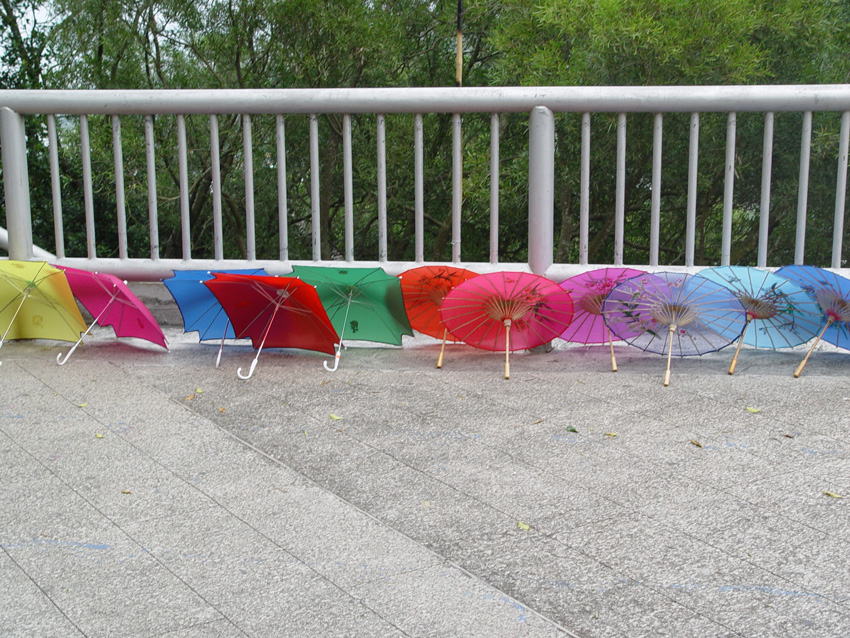The image depicts 11 umbrellas, all open and arranged on a grayish-white concrete or stone patio with rectangular stones. The umbrellas are set in front of a white, dull gray-toned railing with evenly spaced openings, offering a view of the lush greenery beyond. On the left, there are five colorful square-shaped umbrellas in yellow, pink, blue, red, and green. Each of these square umbrellas has a white handle with a J-shaped hook at the bottom. On the right, there are six circular umbrellas featuring intricate oriental prints in shades of blue, purple, pink, and red. These parasol-like umbrellas have straight brown handles without hooks. The precise alignment and vibrant colors of the umbrellas create a striking visual contrast with the muted tones of the patio and railing.